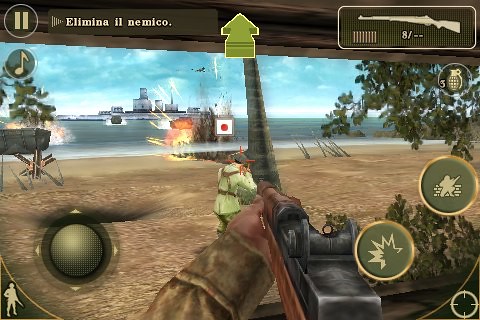This is a screenshot of a first-person shooter video game, capturing the point of view as if the player is holding a long gun, with a visible arm clad in a brown jacket. The scene unfolds on a vast, sand-colored terrain with scattered sticks or debris, and a single enemy target in the distance wearing a beige jacket and appearing to shoot at something unseen ahead. The player's crosshairs are aimed at the enemy's head, indicating they are the focus. Far off in the background, a Chinese flag waves near some explosions and fires, suggesting recent combat activity. Beyond the skirmish area, the ocean stretches with a large boat visible on the horizon.

The in-game heads-up display (HUD) presents various controls and status indicators. In the upper left, a Spanish command, "elimina el nemico," instructs to eliminate the enemy. A pause button and other navigational indicators flank the screen; a round button on the left possibly signifies movement, while the right displays two green directional buttons. Additionally, there is an aiming reticle representing a scope, and three hand grenades within a circular icon at the top. The lower corners of the screen feature curved lines, with small icons likely corresponding to game features or status indicators, including a soldier figure on the left and targeting elements on the right.